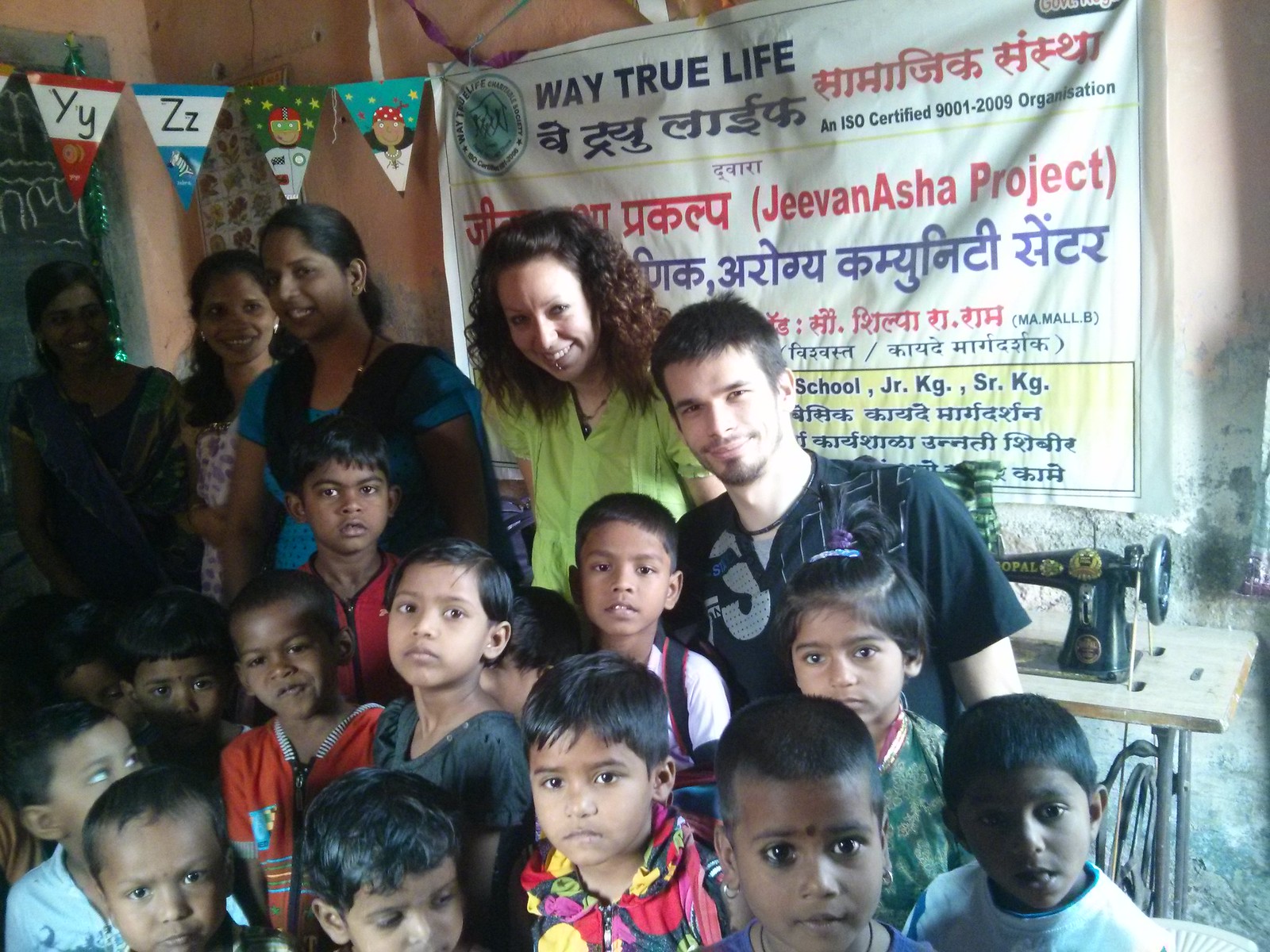In this detailed group photograph, we see approximately 14 South Asian children standing in two rows, with about six children per row and one additional child positioned separately. They are accompanied by a mix of adults, including one Caucasian man and one Caucasian woman, positioned centrally. To their left, there are three South Asian women. The setting appears to be somewhere in South Asia, as indicated by the presence of a multilingual banner in the background. The banner prominently displays "Way True Life" and "Jeevan Asha Project" in English, alongside several scripts in Hindi and possibly other local languages. The banner also mentions that the organization is ISO Certified 9001-2009. Additional details include decorative flags with letters like "YY" and "ZZ," as well as small face illustrations. In the background, behind the group, there's a small desk that appears to have a sewing machine on it. The scene captures a sense of community and shared purpose among the diverse group of adults and children.